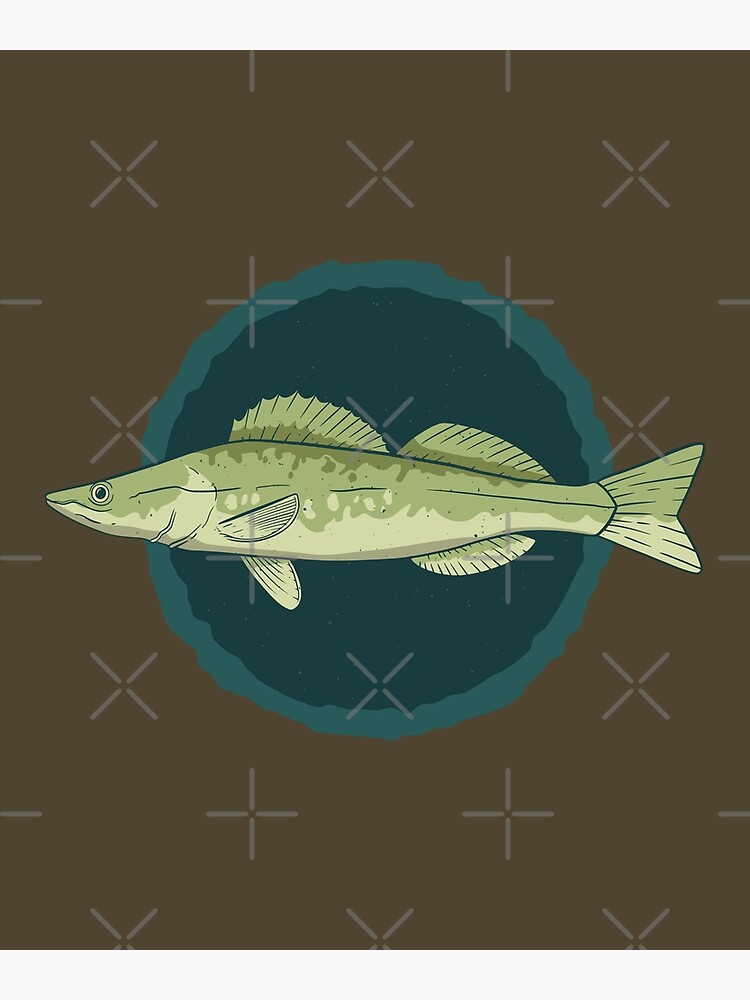This digital illustration features a slender, green walleye fish displayed in a side profile, extending from right to left across the screen. The fish is predominantly a darker green on top, tapering down to a lighter green underbelly, and adorned with dark green speckles. Its head tapers into a distinct point. The fish's dorsal fin has a serrated appearance, while the other fins are smooth. The creature is set against a striking backdrop: a rough-edged, dark teal or blue circle with a lighter blue or green border. This circular element is placed on a brown background, which is intricately decorated with patterns of X's and plus signs.